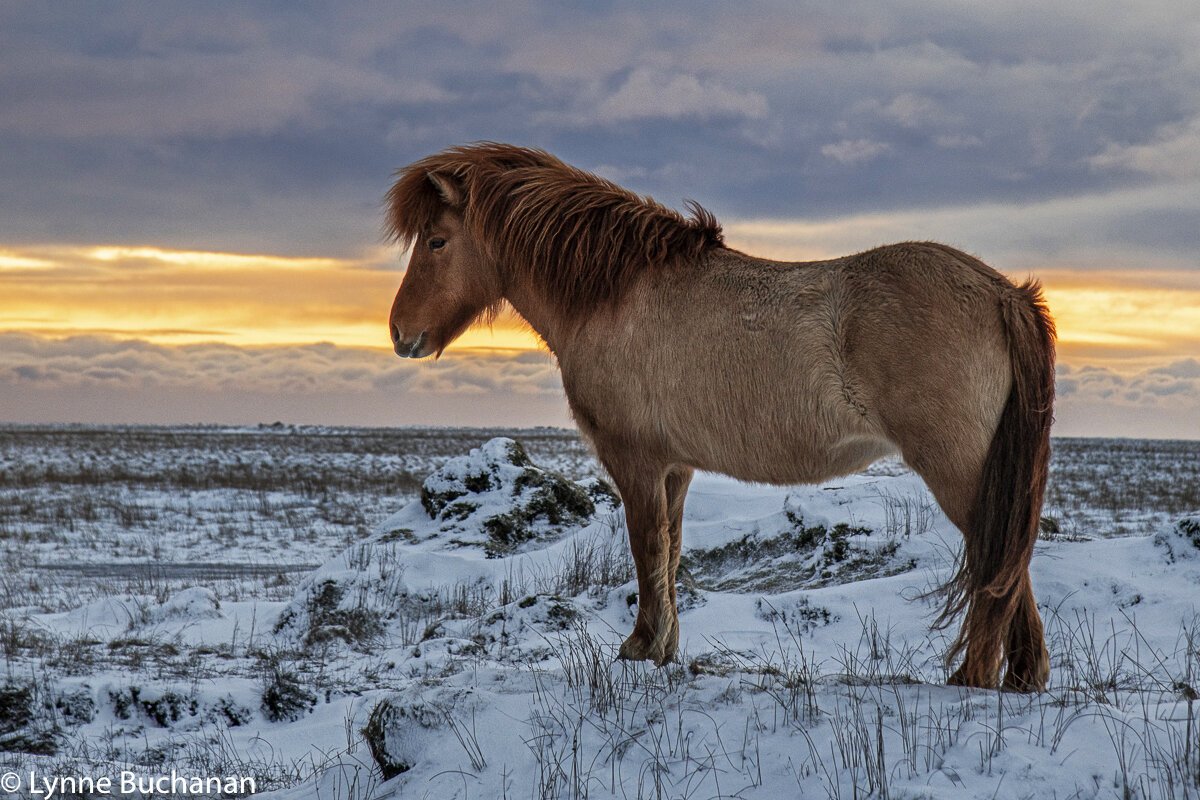The photograph captures a unique wild horse, resembling a miniature or Icelandic breed, standing in the center of a snow-covered, rural landscape. The brown horse features a very thick, dark brown mane that extends from its neck to its head, and an equally thick, dark brown tail. Facing the left, the horse is positioned on a terrain scattered with dark brown rocks and scraggly vegetation interspersed with large patches of white snow. The backdrop showcases a dramatic sky filled with dark gray clouds, with a golden-yellow and orange hue at the horizon, indicating either sunrise or sunset. In the bottom left corner of the photograph, "Lynn Buchanan" and a copyright symbol are inscribed in white text.